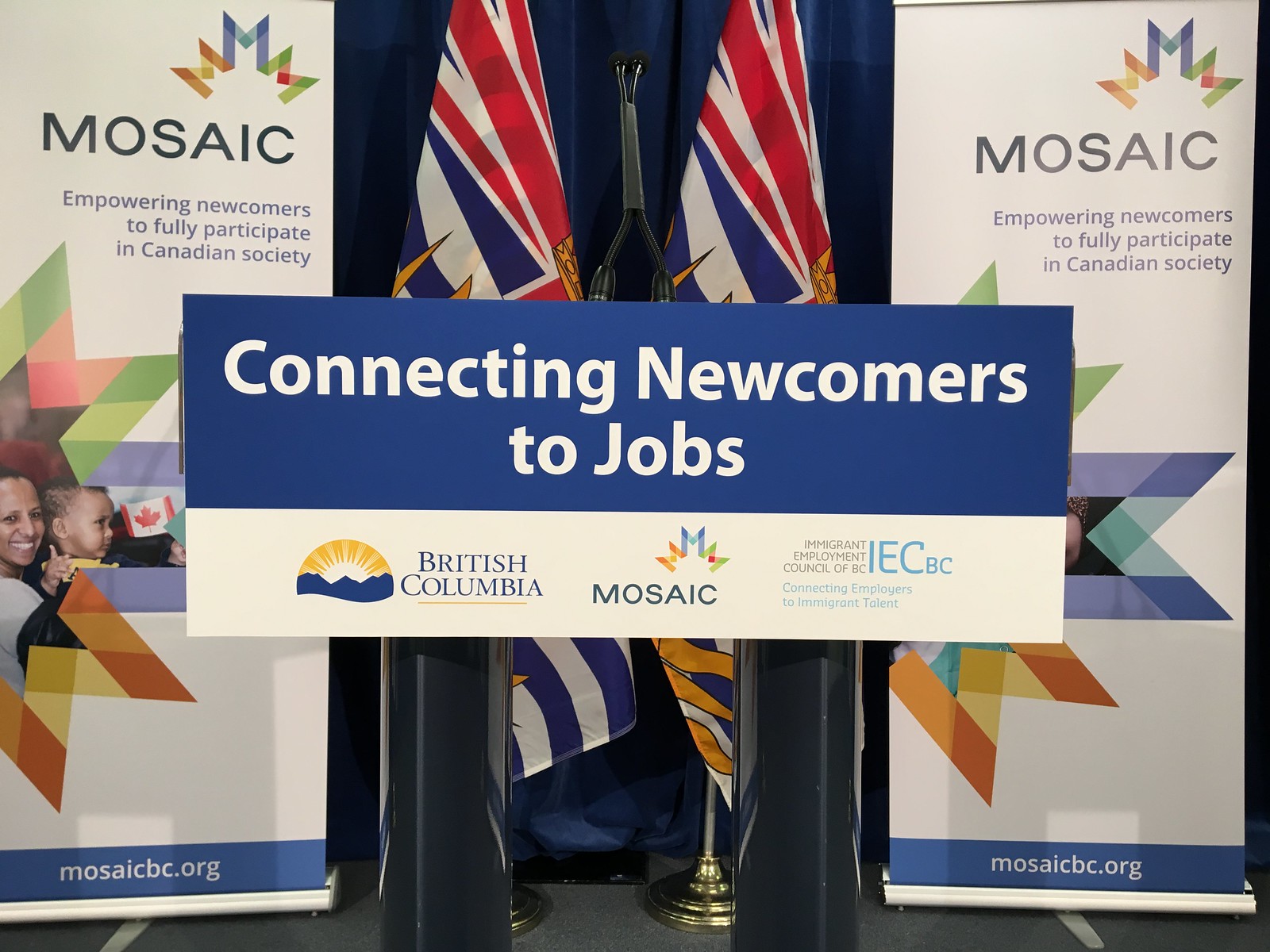The image is a full-color photograph featuring a prominently placed advertisement. At the forefront is a rectangular sign with a dark blue top half, inscribed with the white text "Connecting Newcomers to Jobs." The bottom half of the sign is white, displaying the logos and names of three sponsors: British Columbia, Mosaic, and the Immigrant Employment Council of B.C. (IECBC). The logo of Mosaic appears on two tall white banners that flank the sign on both sides, each bearing the text "Empowering Newcomers to Fully Participate in Canadian Society" in blue font, along with the website "mosaicbc.org" in white against a blue bar at the bottom. Behind the sign and between the banners are two folded flags featuring red, white, blue, and some gold elements, though their exact designs are indistinguishable. The left banner includes an additional graphic of a mother holding her son, who is waving a Canadian flag. The scene is set against what seems to be a stage area.